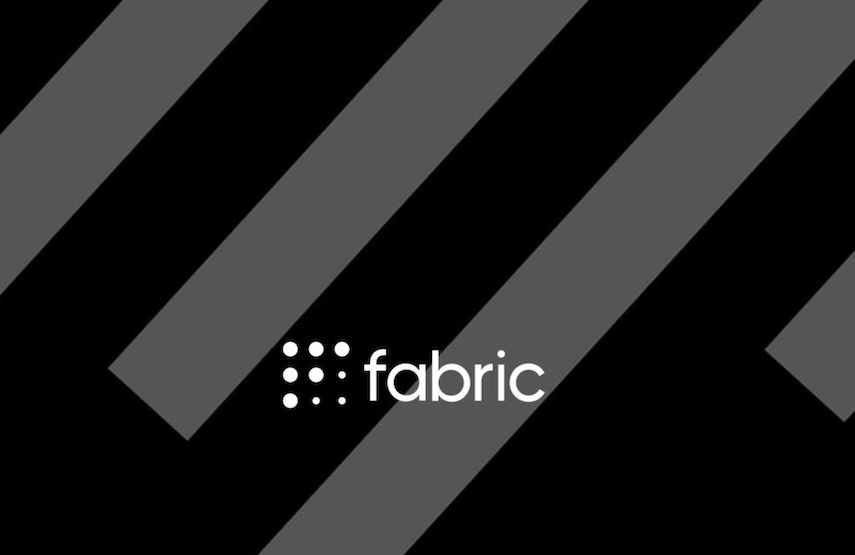The image showcases a distinctive brand logo set against a black background with four barely visible diagonal gray stripes. The logo comprises the word "fabric" written in lowercase white letters, positioned slightly off-center towards the bottom of the image. To the left of the text "fabric," there are nine white circular dots arranged in a 3x3 grid. The top row and the first two dots of the second row, along with the first dot of the bottom row, are large and uniformly sized. The third dot in the second row and the last two dots in the bottom row are smaller in size. The combination of bold and thinner elements, along with the strategic positioning and variation in dot sizes, creates a visually striking and balanced composition.